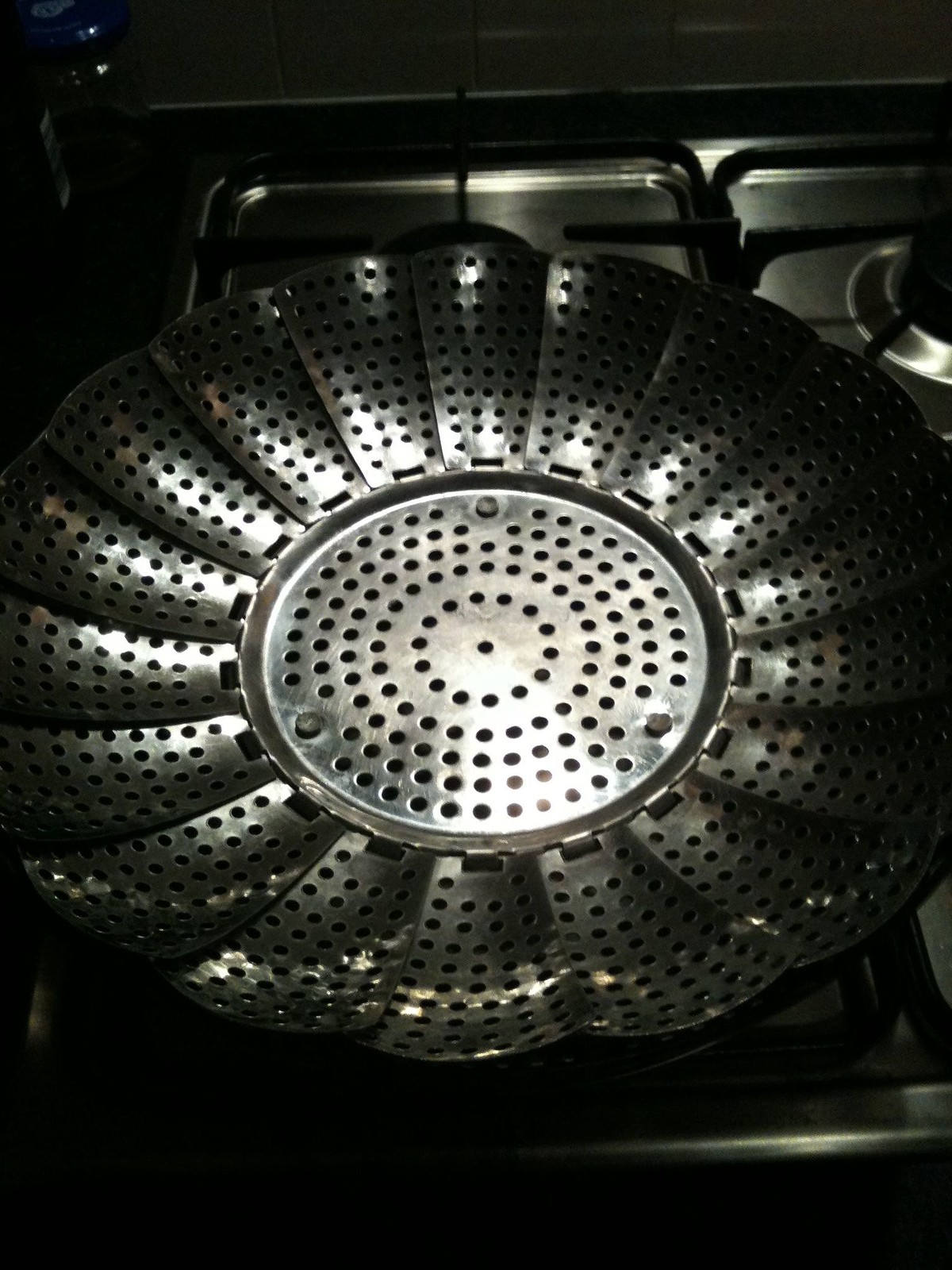This is an extremely detailed close-up image of a large, round stainless steel kitchen colander. The colander has a slightly flattened shape with an intricate design. The edges feature a series of petal-like shapes resembling gas pedals, each adorned with vertical rows of minuscule black holes forming a ring around the colander. The central section is distinctly circular, highlighted by three gray dots, and further decorated with concentric rows of small black holes leading towards the center. The colander is positioned on a gray or black oven burner, with another similar colander visible in the background to the right. The backdrop is predominantly black, accentuating the colander's shiny, silver surface. This design is not just aesthetic but functional, making it perfect for rinsing large vegetables or fruits such as carrots, tomatoes, apples, grapes, cherries, and strawberries.